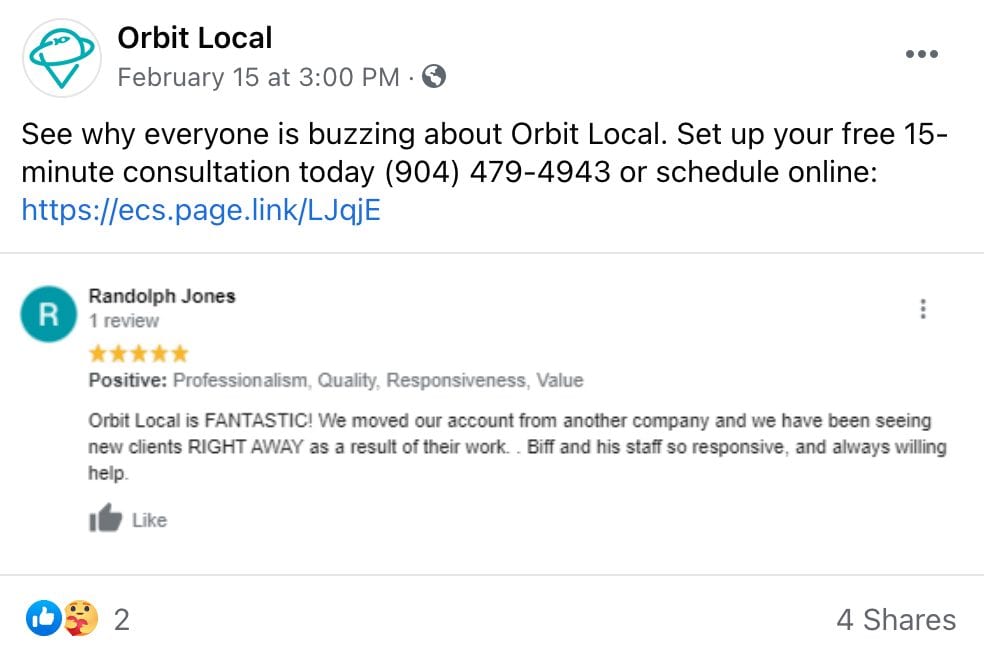Orbit Local recently posted a tweet inviting users to discover why their services are generating so much excitement. They offer a free 15-minute consultation, which can be scheduled via phone or online through an included link. Accompanying the post is a review from Randolph Jones, praising Orbit Local for their exceptional service. Jones mentions that after switching their account from another company, they started seeing new clients almost immediately thanks to Biff and his team, who are described as responsive and always willing to help. The tweet has received minimal engagement, with one or two likes and four shares. The overall design features a white background with black text, and the content primarily consists of customer feedback enhancing the credibility of Orbit Local's client acquisition services.